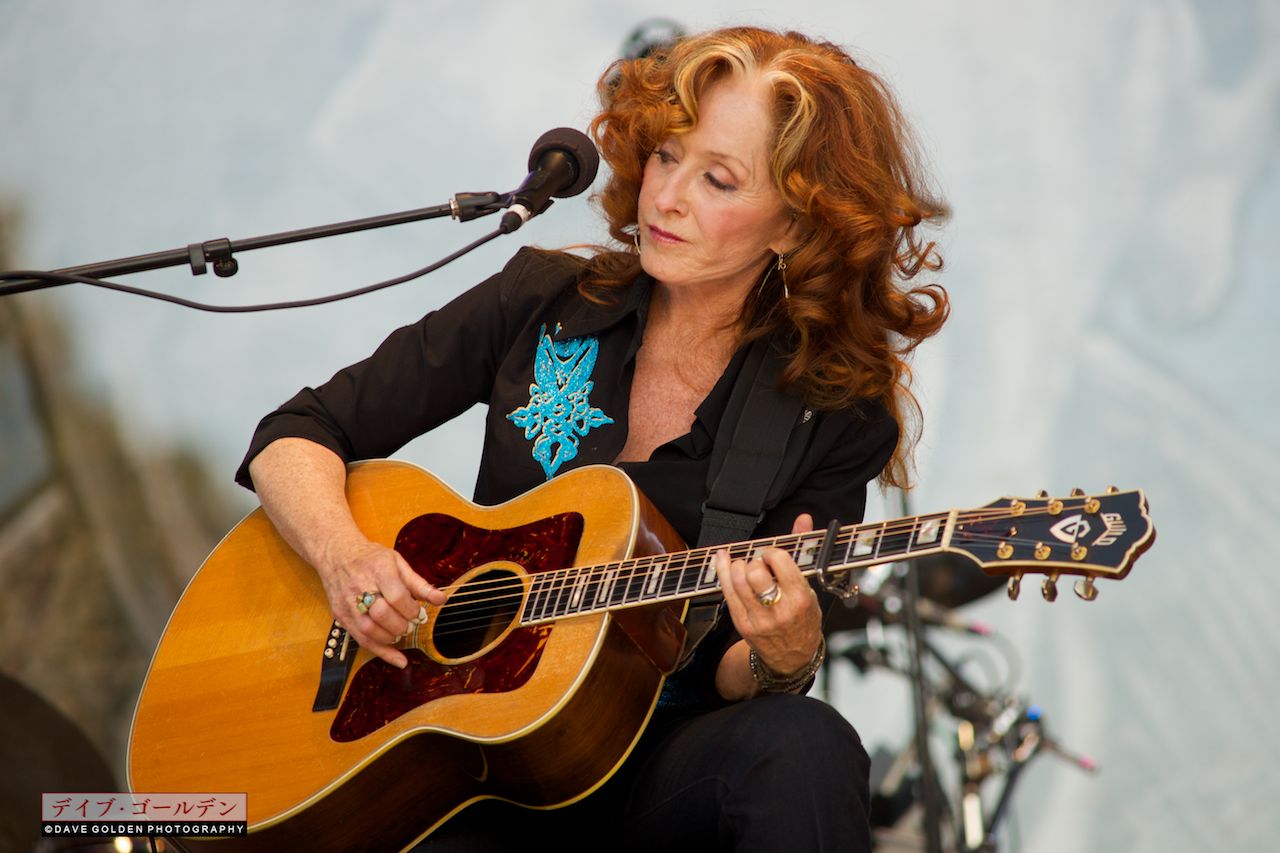In this photograph, the renowned singer Bonnie Raitt is the focal point, captured mid-performance while seated and strumming a light brown acoustic guitar with dark brown accents and gold pegs. Her distinctive curly red hair frames her face as she looks towards the left side of the image, exuding an air of concentration. She is clad in a black shirt adorned with a blue graphic, black pants, and a turquoise-emblazoned guitar strap draped over her shoulders. Small dangly earrings, several rings on her fingers, and bracelets on her wrists add a touch of elegance to her ensemble. A black microphone is positioned from the left side of the frame towards her mouth, indicating she is likely singing or preparing to sing. The setting is well-lit with a white, slightly blurry background that includes other instruments towards the bottom, highlighting Bonnie Raitt in clear and detailed focus.